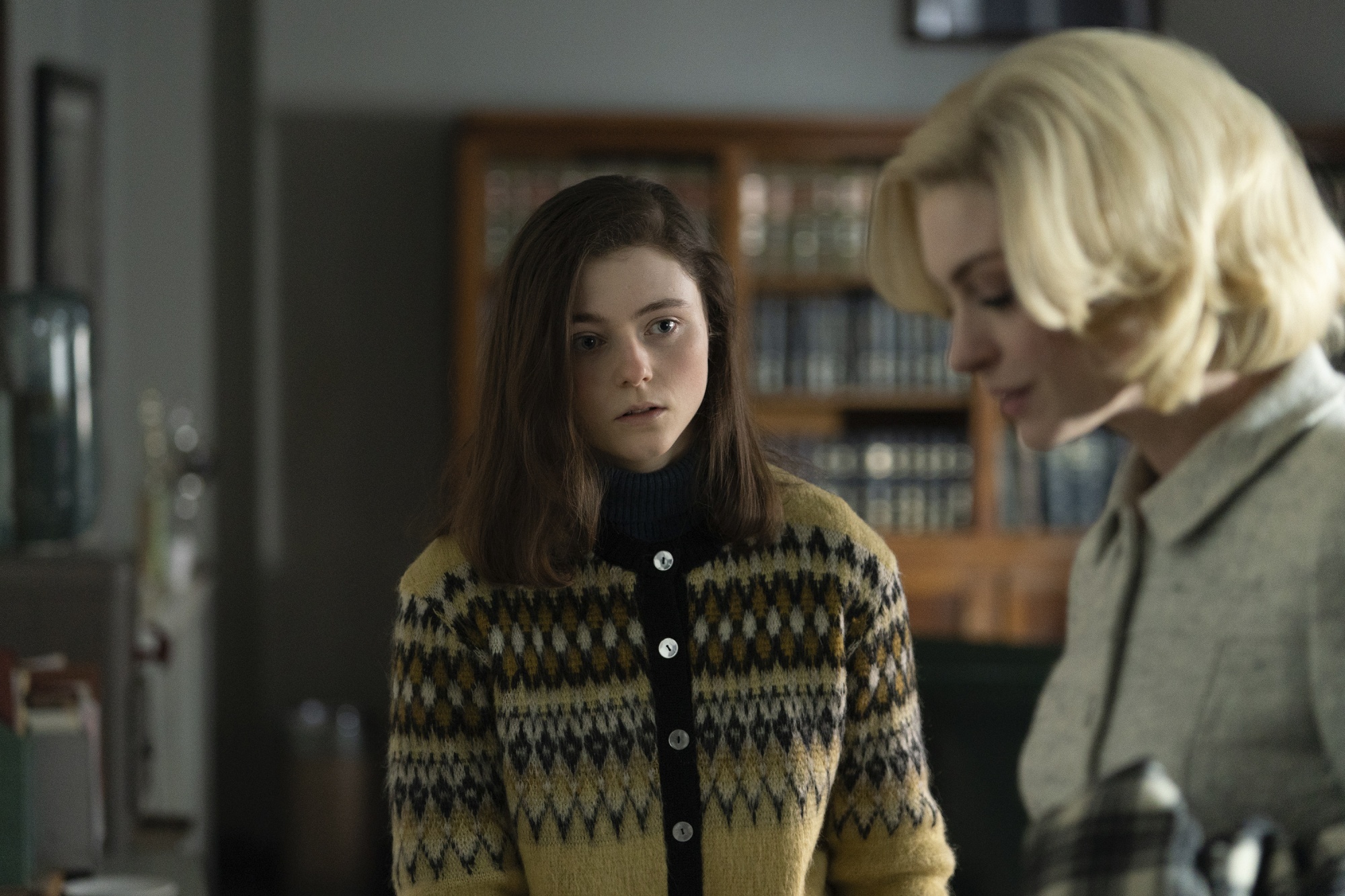In this photo, two women are in a living area with muted colors. The scene captures a moment of tension. The younger woman, likely in her late teens to early twenties, has shoulder-length brown hair and is wearing a tan button-up knit sweater with some designs. She is gazing intently at the other woman, her expression suggesting she is awaiting a response or reaction to an unspoken question. The second woman, who seems to be in her thirties, has chin-length blonde hair and is dressed in a gray collared shirt. Her eyes are downcast, and her face is mostly expressionless. They are positioned waist-up in the frame, with a background featuring blurry, indistinct household items and a prominent wooden bookshelf filled with books. The setting has gray walls and contributes to the overall muted atmosphere of the image. The younger woman’s concerned demeanor contrasts with the older woman’s subdued, almost detached appearance, adding depth to the scene.